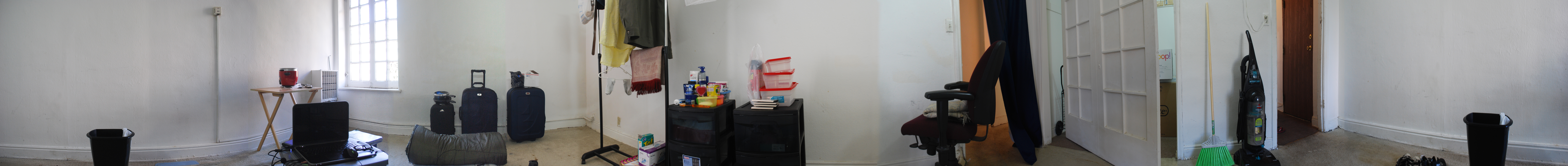The collection features a photograph series depicting various aspects of an unoccupied living space and close-up details of items within the room. 

The primary image exhibits an almost empty room with limited furniture, predominantly a modest coffee table. The secondary composite image unfolds across four distinct snapshots: 

1. The first snapshot reveals a trio of black, wheeled suitcases, accompanied by a foldable coffee table and a black trash can, placed against the backdrop of a window. Additionally, a rolling clothing rack adorned with a few garments is observable.
2. The second snapshot focuses on a dresser cluttered with disposable plastic dishware, while a black rolling office chair stands nearby.
3. The third and fourth snapshots blend together visually, featuring a black vacuum cleaner, the aforementioned black trash can, several indistinguishable items on the floor, and a broom with a white handle and green bristles. 

Each image captures the essence of a disorganized, sparsely-furnished room awaiting occupancy or arrangement.